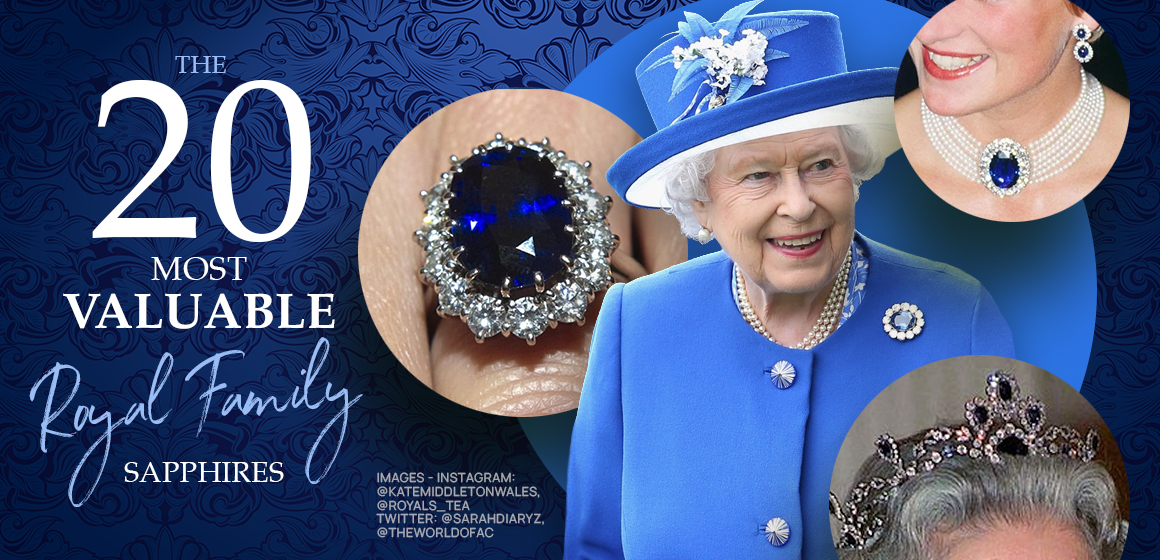This image gives off the vibe of an advertisement, highlighting the 20 most valuable royal family sapphires. Centered in the graphic, Queen Elizabeth II is depicted wearing a striking blue outfit, complete with a matching blue hat adorned with white flowers. Her ensemble is complemented by a sapphire brooch pinned to her left breast. The right two-thirds of the image showcases three circular close-ups of different pieces of sapphire jewelry, each surrounded by diamonds. These include a sapphire ring, a sapphire necklace likely belonging to Princess Diana, and a tiara embellished with sapphires. The background features a luxurious blue floral pattern, with credits listed at the bottom for image sources including Instagram accounts like Kate Middleton Wales and Twitter handles like Royals_T. The left side of the image prominently displays the elegant text, "The 20 Most Valuable Royal Family Sapphires."